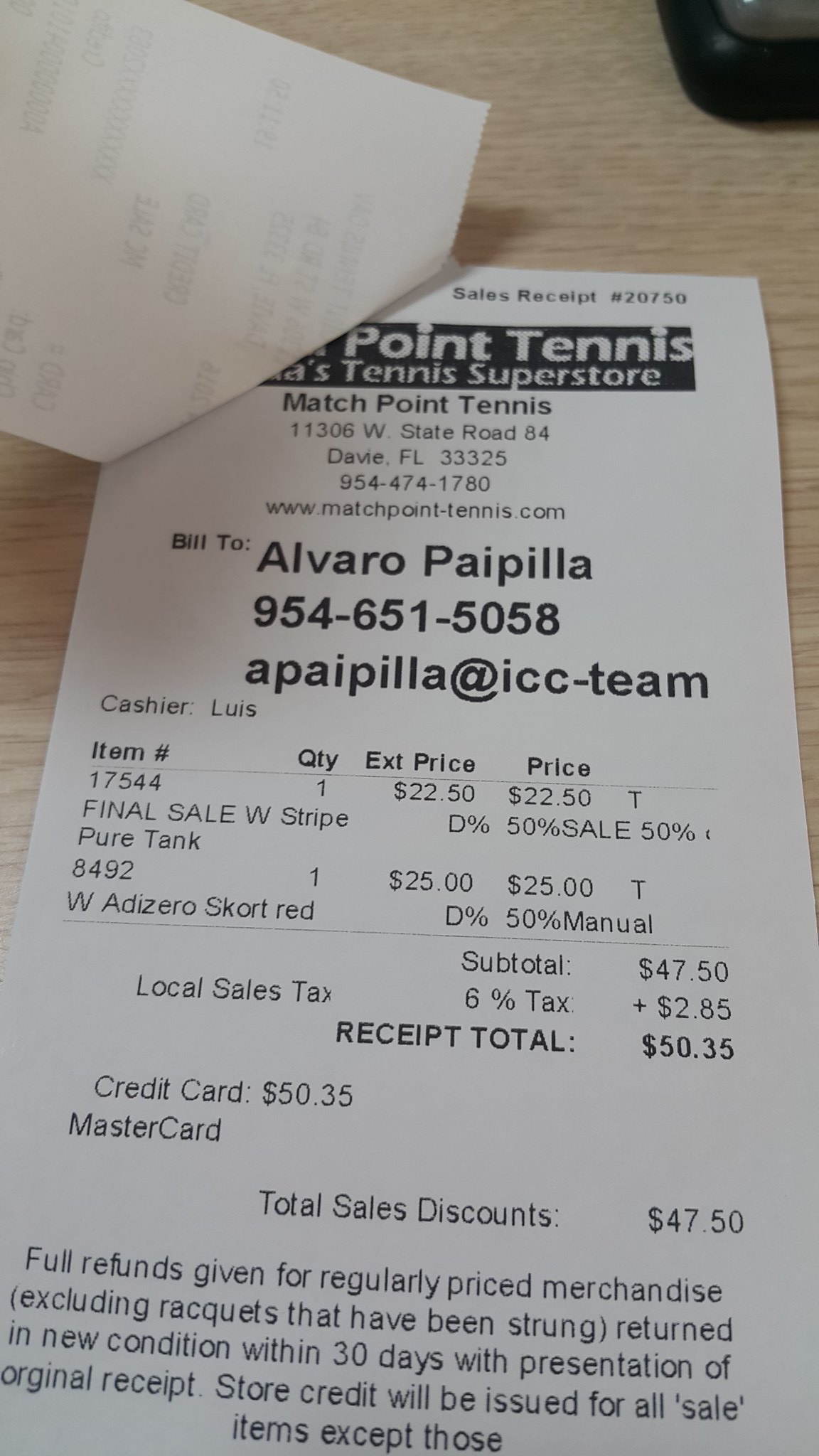The image displays a paper receipt from a retail store named MatchPoint Tennis, a tennis superstore. The store is located at 11306 West State Road 84, Davie, Florida, 33325. Their contact number is (954) 747-1780, and their website is matchpointtennis.com. The receipt is billed to Alvaro Papilla, who can be reached at (954) 651-5058.